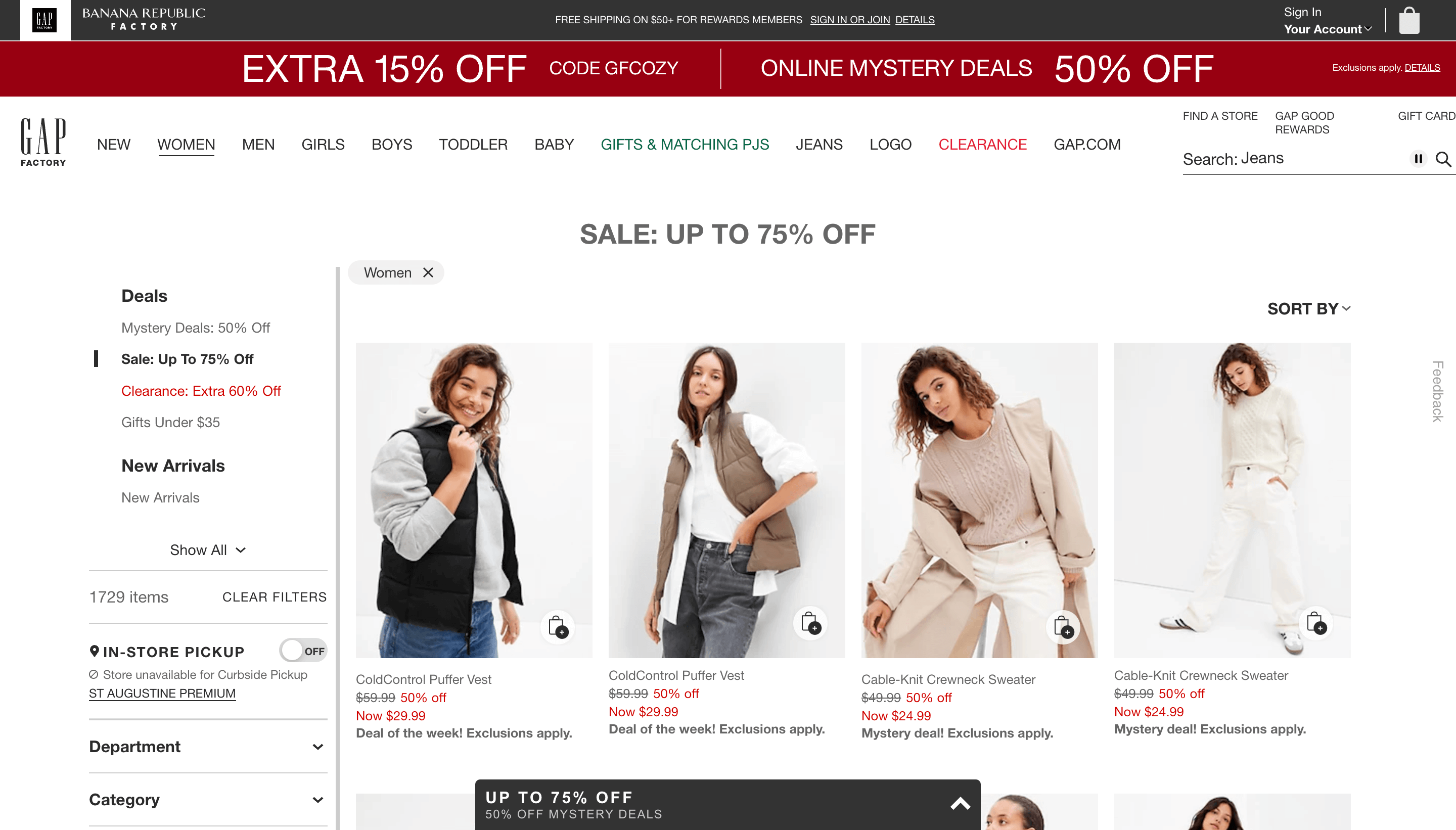Top left corner of the image features a promotional banner for Banana Republic Factory offering free shipping on orders over $50 for rewards members, along with a prompt to sign in or join. Below that, a shipping bag icon is displayed next to red bars indicating an extra 50% off code "GFCOZY" for online mystery deals. Additionally, it highlights details about discounts: 50% off for various categories including women, men, girls, boys, toddlers, and baby products, as well as gift items, metro pajamas, and jeans.

Another segment of the image shows the Banana Republic Factory logo, along with options like "Find Store," "Clearance," and "GF Goods." There's also a search bar with the term "jeans." The left side of the banner lists multiple deals such as an extra 50% off mystery deals, up to 70% off clearance items, and an extra 60% off select merchandise.

Additional highlighted text includes offer details like new arrivals, potential credits of up to $1,729, options to filter and clear selections, store pickup availability, curbside pickup options, and mentions of premium items now priced at $2.99. The assertive call to action "Check it, uh huh, control" suggests an emphasis on taking advantage of these offers promptly.